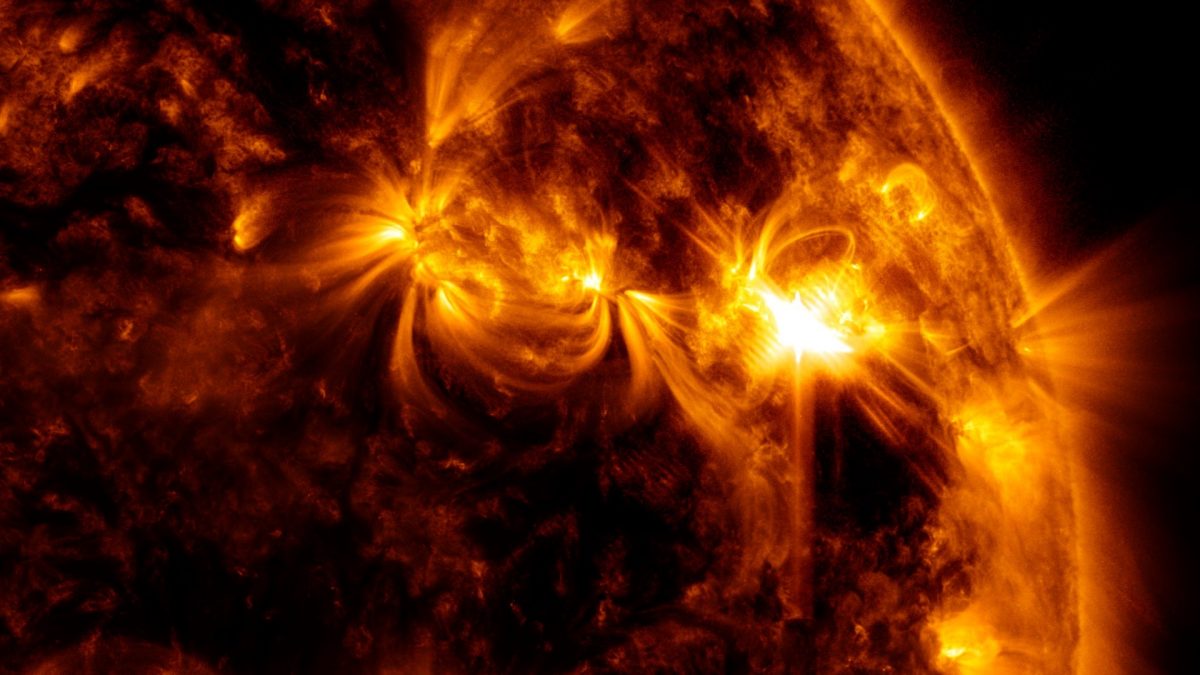The image depicts a section of the sun captured in intense detail, likely through infrared or a specialized visible wavelength filter. The backdrop is a deep, expansive black, representing the emptiness of outer space. At the center, a mesmerizing display of fiery colors—ranging from deep reds and oranges to bright yellows and whites—dominates the scene. This is a striking close-up of the sun, highlighting violent solar activity.

One can observe swirling patterns of light within the sun's surface, reminiscent of solar flares that snake and curl violently, evoking a sense of immense thermonuclear power. These flares and sunspots create a dynamic tapestry of glowing, turbulent plasma. In the image, there are notable contrasts: brighter yellow areas indicative of higher temperatures and darker regions on the left side where the sun's surface appears cooler, displaying darker browns and reds.

Additionally, jets of solar material seem to be spewing from the sun into the empty space, captured brilliantly on the right side of the image. The overall effect is a captivating, almost mesmerizing view of our star, dense with swirling lights and fiery activity, frozen in a moment of cosmic dynamism.